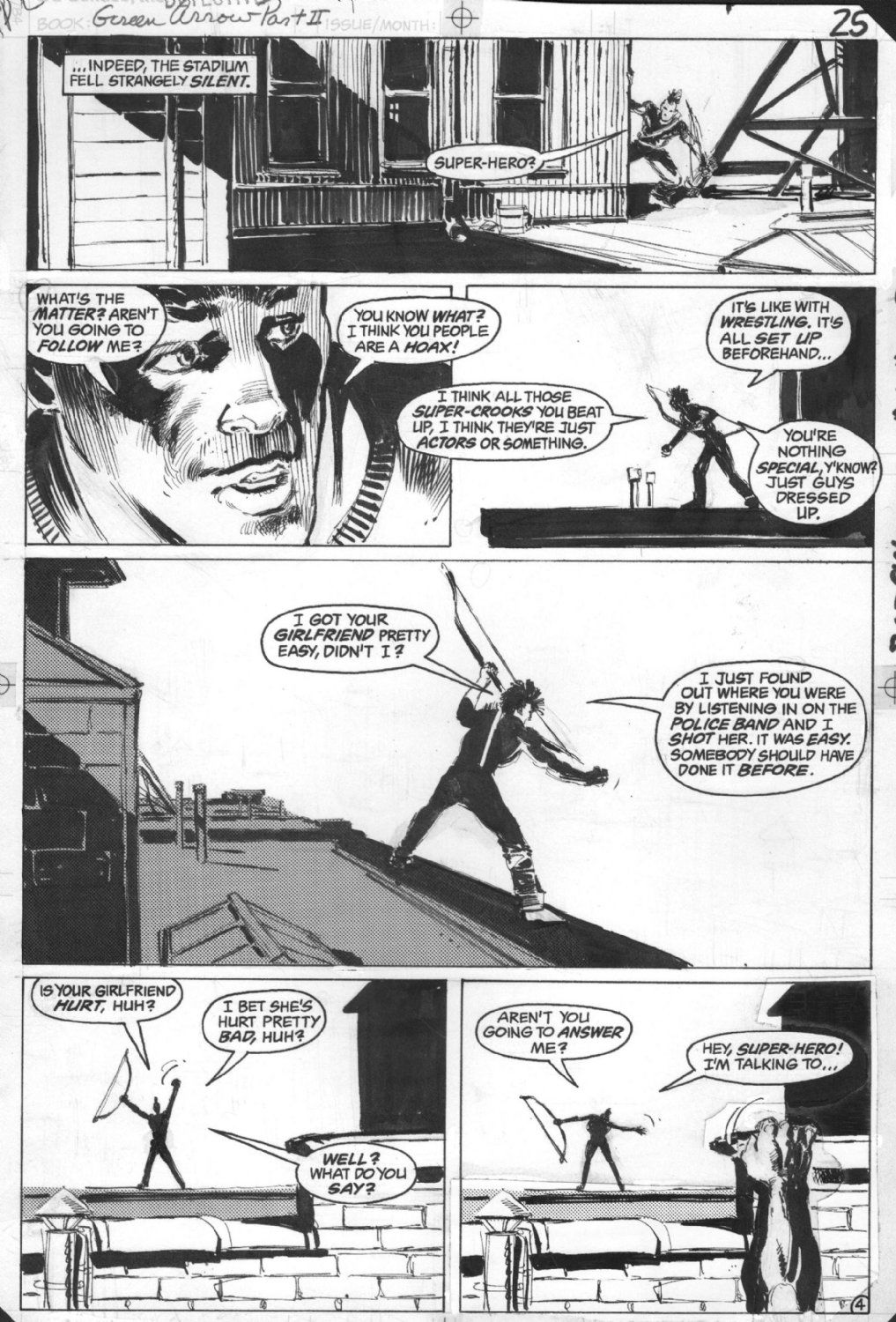The image is a black-and-white scan of an original comic book art page, labeled at the top as "Green Arrow Part Two" in handwritten text. The page is composed of six separate panels arranged in various rectangular and square shapes. The negative space, known as gutters, surrounds these panels. In the top right corner, the number "25" suggests this might be page 25, while a small circled "4" in the bottom right corner could indicate additional information about the page's sequence.

The narrative within the panels unfolds an intense rooftop confrontation involving a person with a bow and arrow. Each panel features dialogue and text that drives the story forward. The first panel depicts an old building with someone peeking around the corner, engaging in a dialogue that begins with a mysterious statement: "Indeed the stadium fell strangely silent, siren." The hidden figure taunts with the word "superhero."

A close-up of a face in the next panel reads, "What's the matter? Aren't you going to follow me? I think you people are a hoax." Subsequent panels reveal the same character with a bow and arrow, walking to the side while continuing a cynical monologue: "I think all those super crooks you beat up are just actors, like wrestling. It's all set up. You're nothing special, just guys dressed up."

The tension escalates as the archer claims to have easily located and harmed the superhero's girlfriend by eavesdropping on the police band, boasting about shooting her. In another panel, the archer, positioned on the side of the roof with his hands raised and his arrow drawn, taunts, "Is your girlfriend hurt? I bet she's hurt pretty bad. What do you say?"

The final panels depict the archer continuing his taunts, asking, "Aren't you going to answer me?" as he provocatively insists, "Hey superhero, I'm talking to you." The page ends with this unresolved confrontation, captured entirely in black and white, emphasizing the dramatic tension inherent in the storyline.